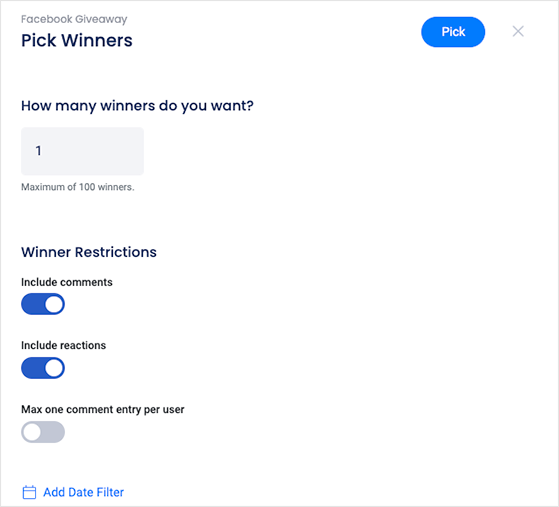The image features a user interface for a Facebook Giveaway, set against a solid white background with light gray outlines. In the upper left corner, small gray text reads "Facebook Giveaway," while below it in bold, black text is the prompt "Pick Winners." 

On the upper right side, there is a blue oblong action button with white text that says "Pick," adjacent to a small gray "X" icon. 

Underneath, in small black text, a question asks, "How Many Winners Do You Want?" This is followed by a white box containing the number "1," with the note "Maximum of 100 Winners" written beneath. 

Further down, in bold text, the section "Winner Restrictions" includes various options: "Include Comments" with a blue toggle button that is turned on, "Include Reactions" also with a blue toggle button that is turned on, and "Max 1 Comment Entry Per User" which has a blue toggle button that is not turned on.

At the bottom, there is a small blue calendar icon accompanied by blue text that reads "Add Date Filter."